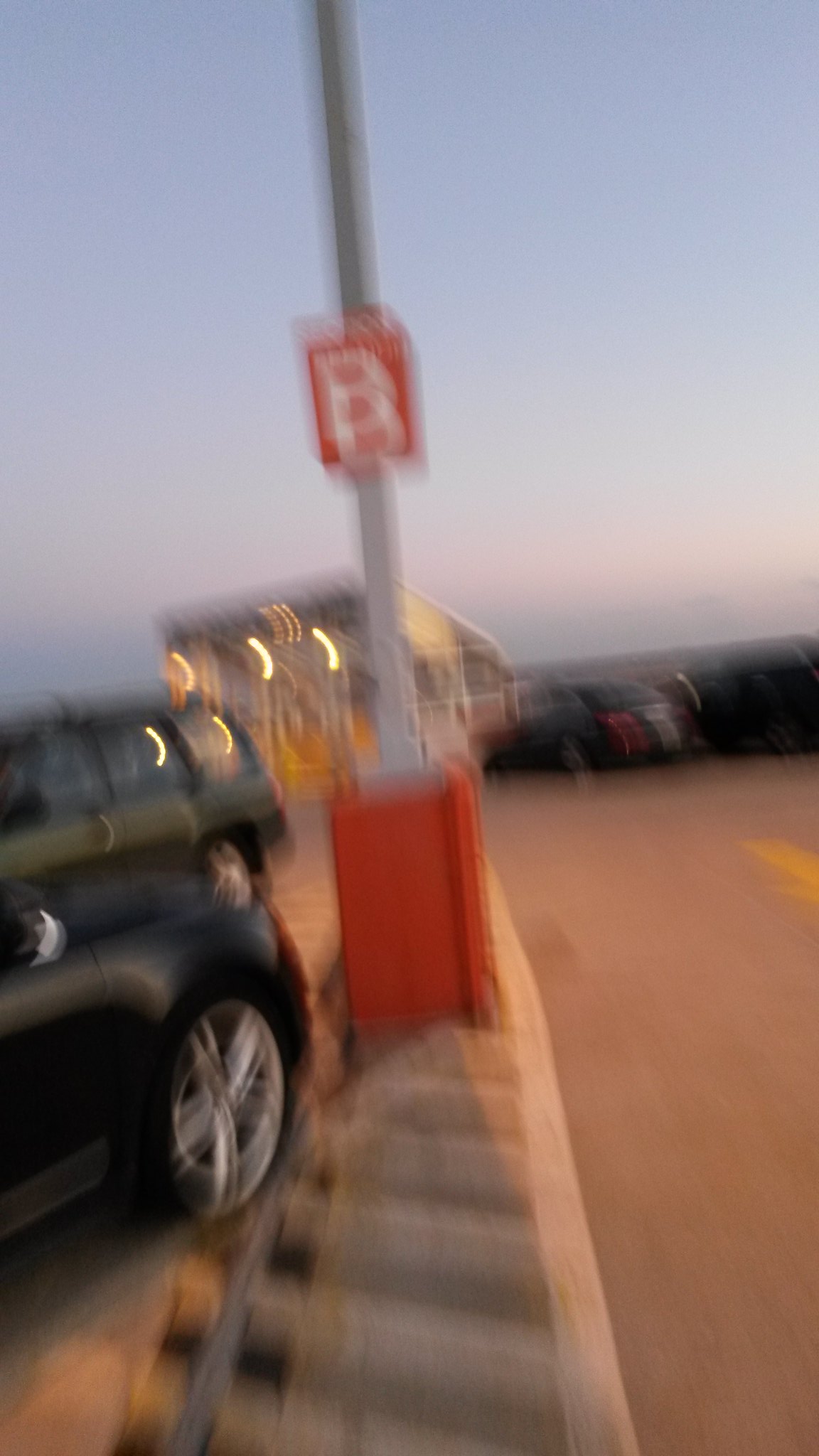A blurry image captures a rooftop parking lot scene. The lot features a central median running from the bottom center of the frame to the midpoint, adorned with a white line on its right side and horizontal cross stripes. The median ends in a red cement square at its top, from which a steel pole rises out of the frame. Atop the pole, a square box with the letter "B" in white stands out against the red background. To the left of the pole, two cars are diagonally parked: one appears to be the front end of a black car, while behind it, a green station wagon has its engine facing outwards with its rear against the median. A small structure, possibly the top of a stairway with a canopy, is visible behind the pole, suggesting this is a rooftop garage. The background features a clear blue sky that spans the entire width of the image.